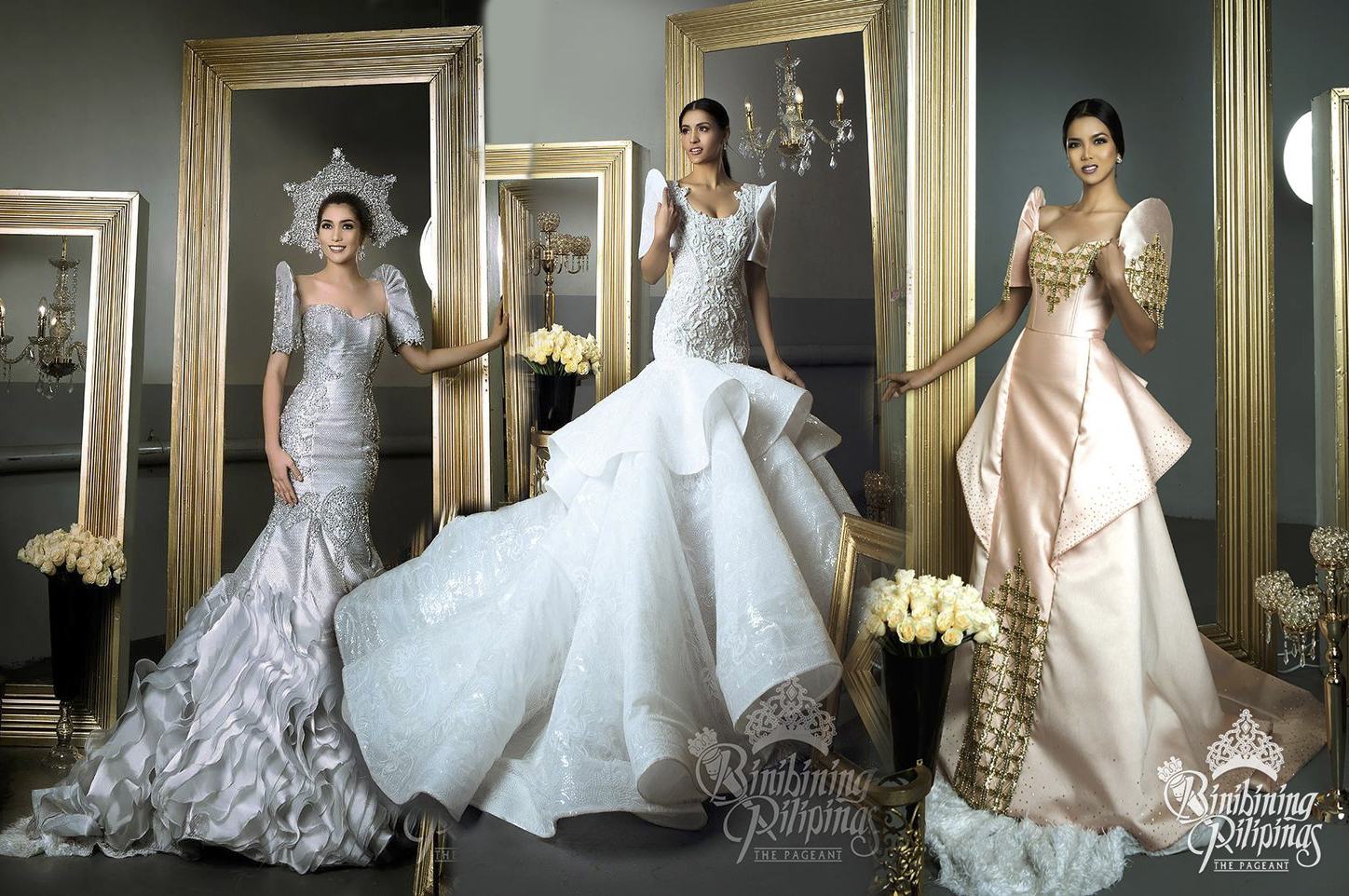In this striking advertisement for wedding dresses, three dark-haired women pose elegantly in front of tall, ornate mirrors with elaborate gold-patterned borders. The leftmost woman dazzles in a silver dress with puffed upper sleeves and an extravagant frilly train that cascades to the floor, resembling flowing hair. Adorning her head is a unique star halo. The central figure wears a traditional white wedding gown with intricate patterns and multiple layers, fanning out generously at the bottom in ruffled splendor. Completing the trio, the woman on the right dons a peach wedding dress with gold accents, including an ornate shoulder detail and sections that draw attention to her silhouette. The setting is opulent, featuring chandeliers and suggesting a pageant-like atmosphere, perfectly capturing the grandeur and elegance of bridal fashion. The smiles on all three women add to the overall enchanting visual, making this advertisement a captivating showcase of wedding attire.